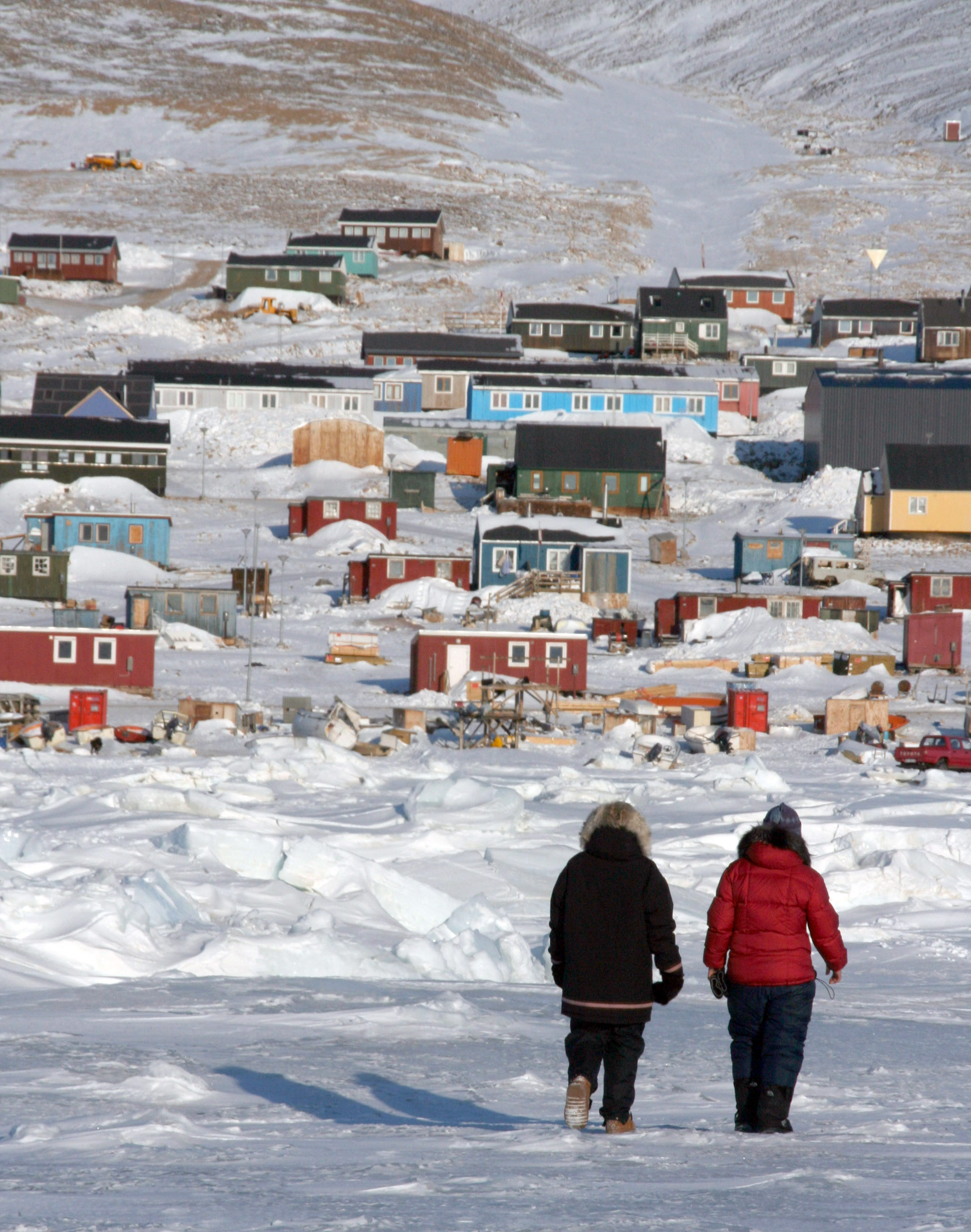A vibrant winter scene captures a neighborhood of colorful, one-story mobile homes nestled amidst a snow-covered landscape. The image, in portrait mode, shows a variety of house colors—red, green, light blue, yellow, white, and orange—against the backdrop of snow-covered hills that span from the top left to the top right of the photo. In the top-left corner, there's an excavated area where the snow appears notably deep. The valley between the hills is thick with ice and partially melted snow. 

In the foreground, two people, dressed in heavy winter attire, walk across the snowy ground. The person on the left dons a large, fluffy-hooded brown coat with dark brown gloves and tan and white snow-covered shoes. The person on the right wears a red jacket without the hood up, a blue cap, and black boots, holding gloves in their right hand. To the far right of the image, a red car is visible. The vivid colors of the houses and the contrast of the heavy winter clothing against the dense snow create a strikingly detailed winter tableau.